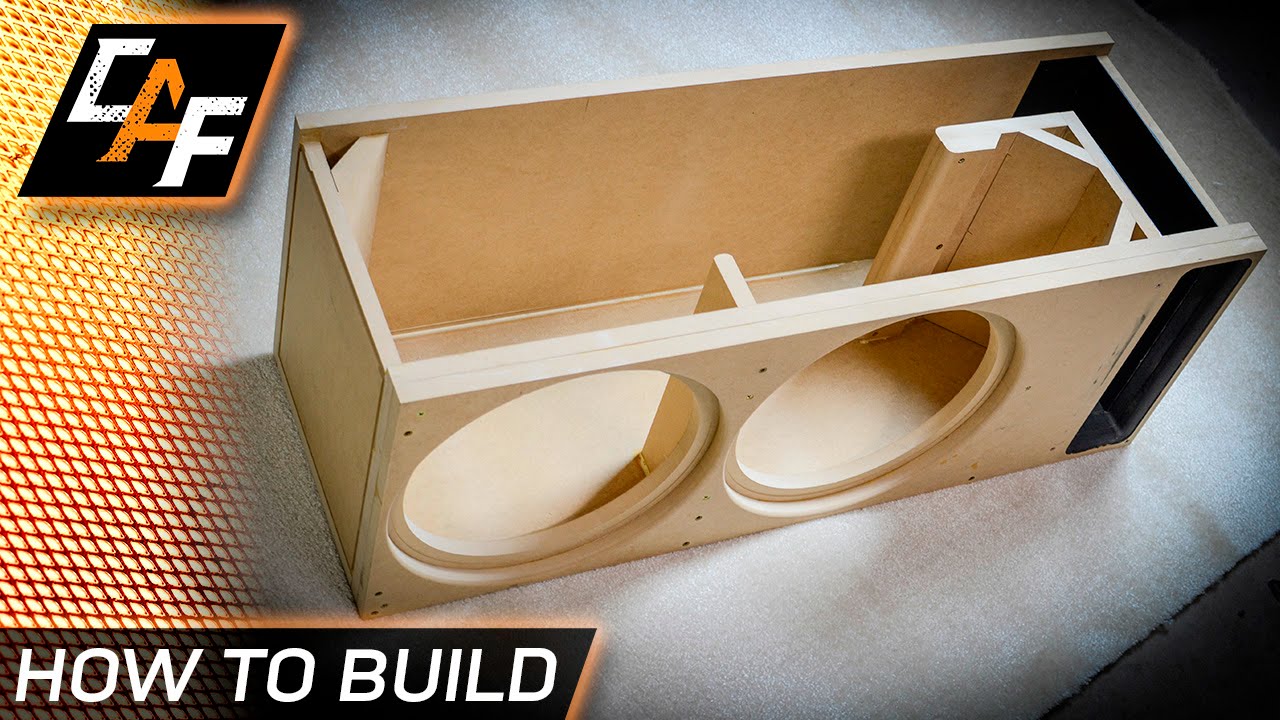This is a photograph of a YouTube video thumbnail. The image features a white table with dark gray muted edges and a wooden box prominently displayed on top. The box is rectangular with three sides and a base, constructed from pine-colored wood. It has two circular holes on the front side, which might be intended for holding cups or speakers. Adjacent to the box on the left side is a gold zigzag piece of fabric. In the bottom left-hand corner of the thumbnail, there's a black square with white text that reads "HOW TO BUILD," outlined in burnt orange. The top left corner displays a design with the letters "CFF," with the middle "F" represented by an orange circle. Overlapping the left-hand side of the box is what seems to be an orange plastic chain link with some holes visible.